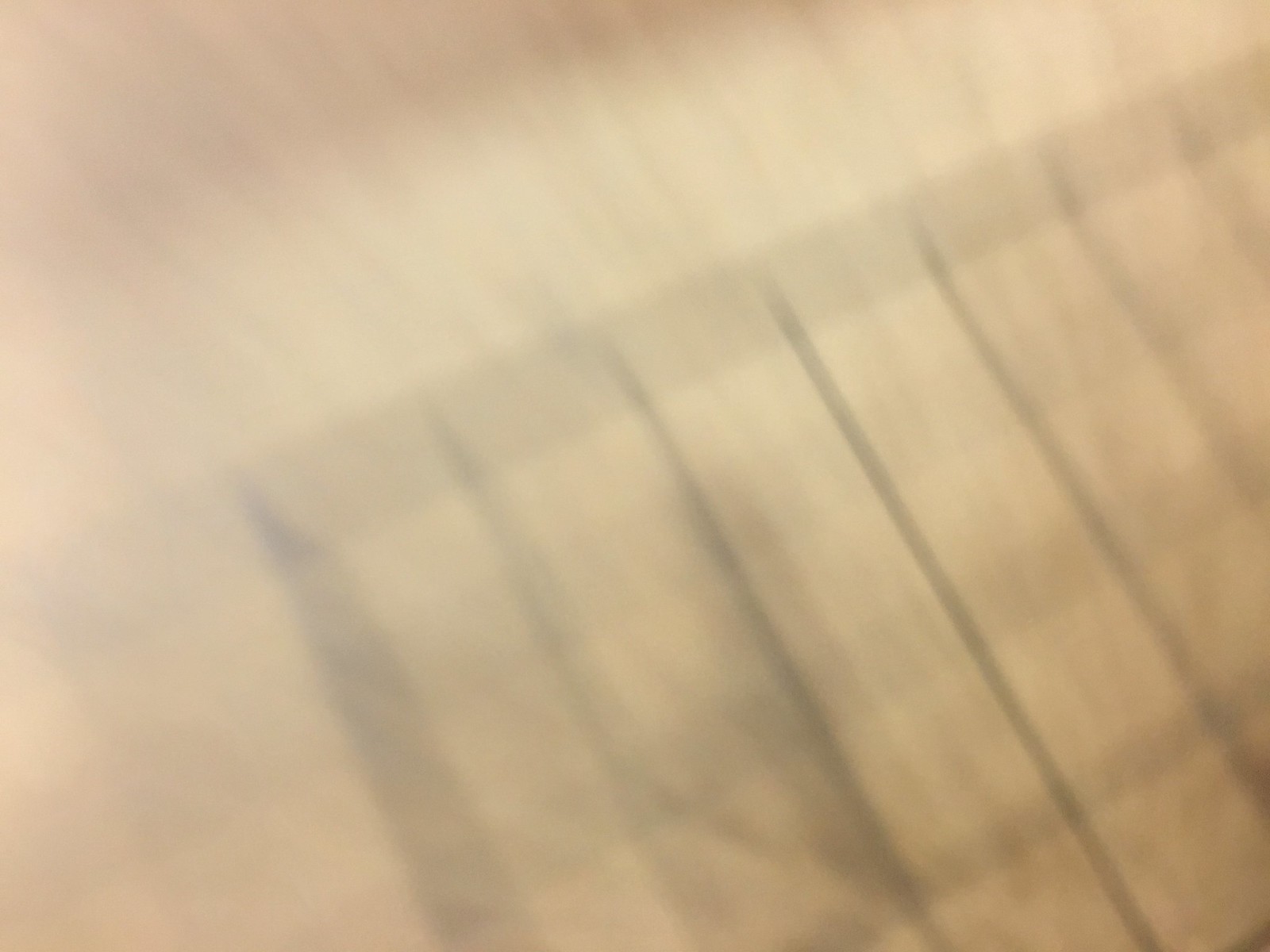Blurry and heavily distorted, this photograph appears to capture a piece of paper with some type of diagram or grid-like structure. The image quality is poor, making it challenging to identify specific details. However, angled towards the bottom right corner, there are several vertical black lines set against a light brown or tan background. These lines intersect with a thicker, barely visible black border, which interestingly extends over the edge at the top of the photo. The pattern resembles either an oven grate or a calendar grid. The overall color palette consists of muted tans and blacks, further complicating clear identification.